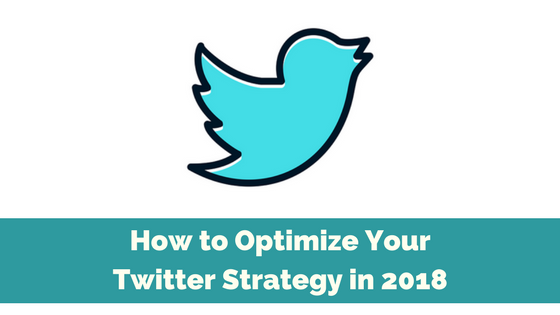At the center of the page, there is an image of the old Twitter logo, which was used before the platform transformed into "X." The logo features a stylized bird in a striking aquamarine color. This bird silhouette is accentuated by a white border, which is particularly visible around the head, beak, tail, and feather tips. Encasing this white border is a thicker black outline. The bird itself is minimalistic, with no facial features or feathering patterns—just a sleek silhouette. The bird appears to be looking slightly upwards to the right, its beak partially open with hints of the white border visible in the small gaps between the beak. Its wings are spread as if in flight, and its belly curves elegantly into the tail area.

The background is plain white, making the logo stand out prominently. About an index finger's width away from the logo, there is a bold, prominent banner. This banner has a teal background and features large, bold, white text that reads "How to Optimize Your Twitter Strategy in 2018." In this text, specific words are capitalized: "How," "Optimize," "Your," "Twitter," and "Strategy." The bird appears to be dynamically poised in mid-air, emphasizing a sense of motion and vitality on the page.